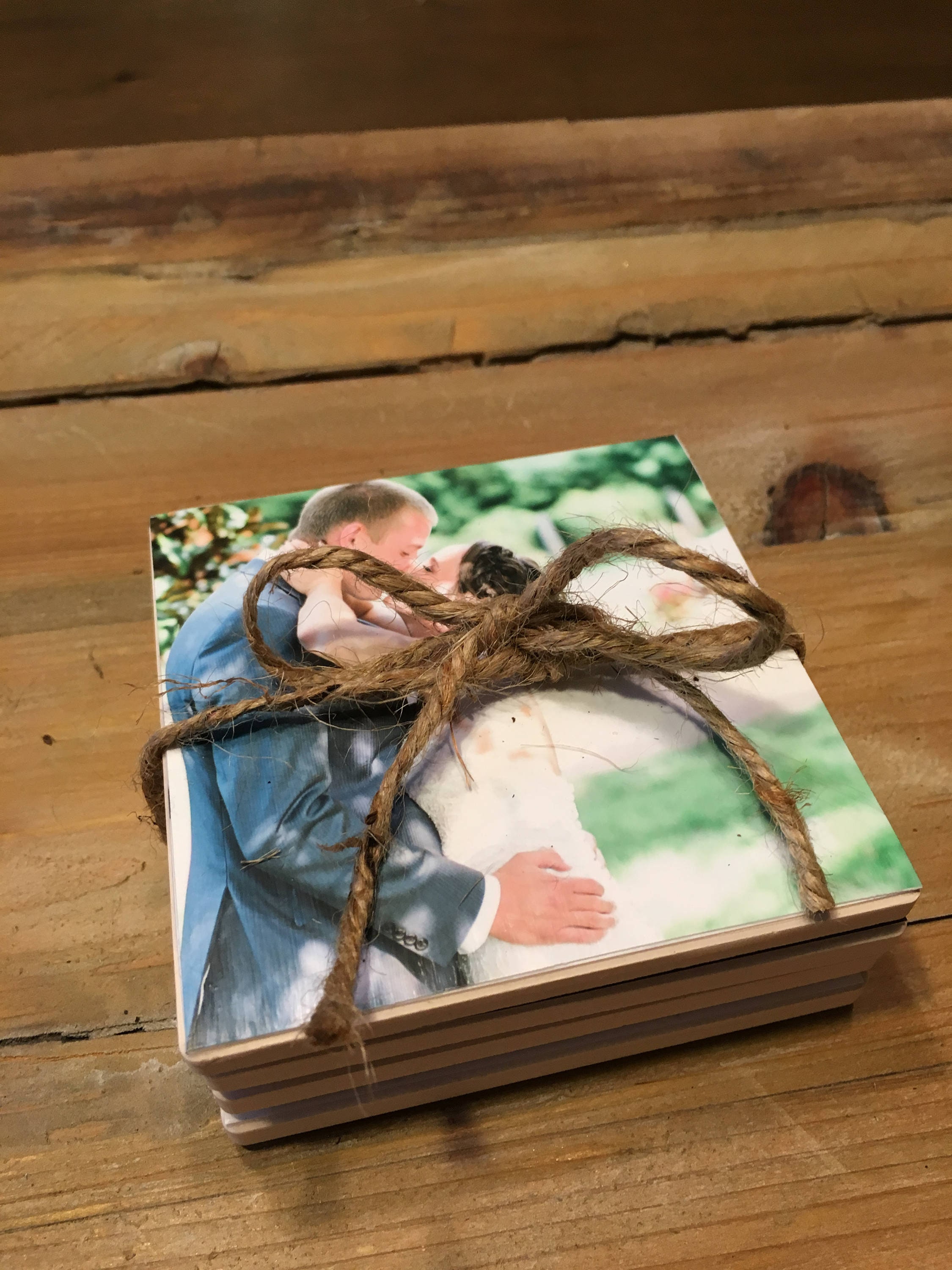The image is a detailed photograph of a stack of custom-made, square-shaped coasters, likely intended as a wedding gift. Each coaster features a glued-on photo of a bride and groom on their wedding day. In the picture, the couple is positioned on the left side of the coaster, kissing passionately. The bride, in a white wedding dress, has her hands wrapped around the groom’s neck, while the groom, dressed in a dark jacket, holds her by the waist. The background of the photo shows a blurred scene of grass and trees, making the couple the sharp focal point. The stack consists of four coasters, tied together with thick, brown twine, arranged in a bow. This quaint bundle rests on a table made of rough, rustic wooden planks, with minimal shadow and an undefined light source.